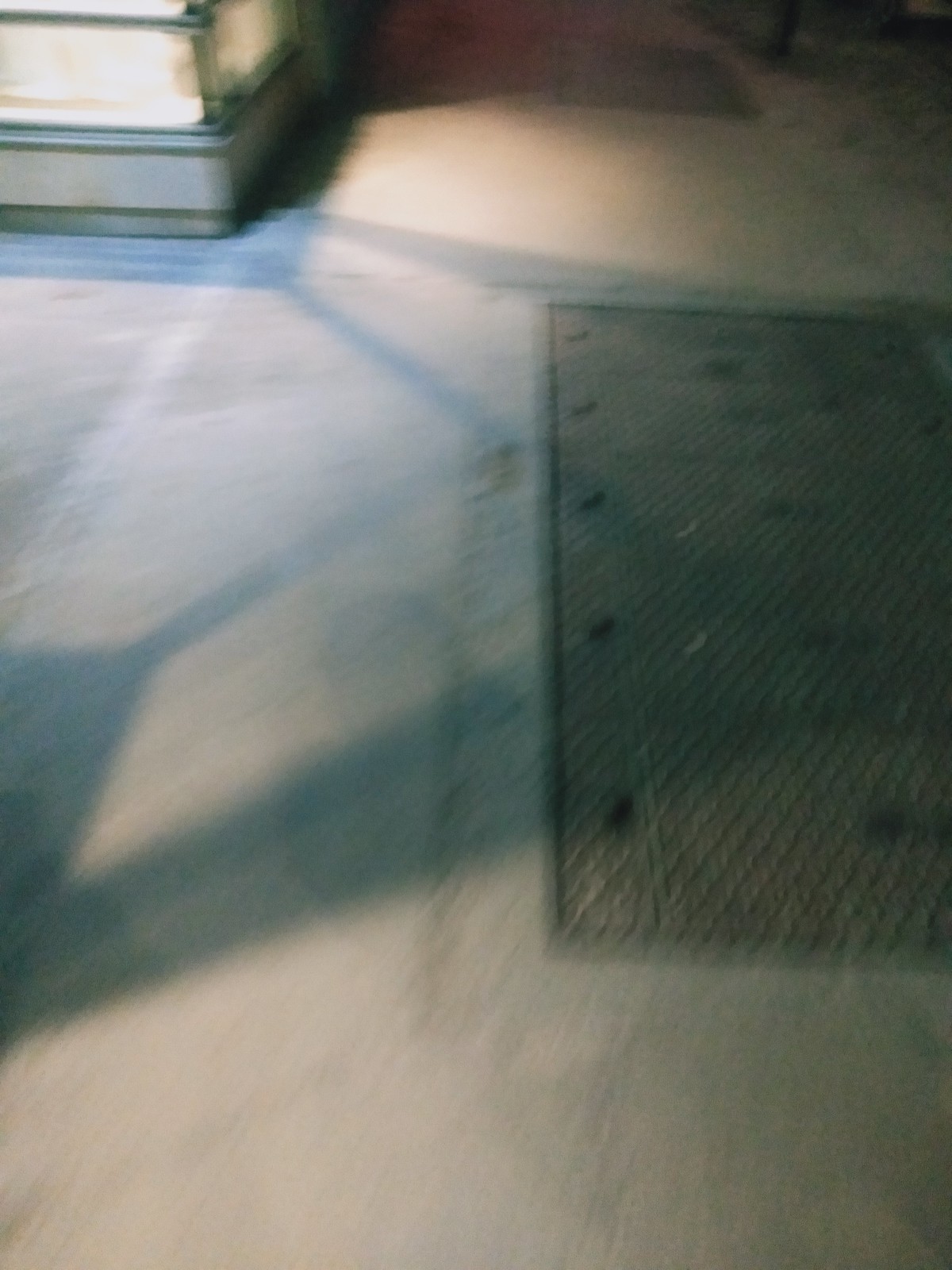The image is a blurry and shadowy nighttime scene, most likely of a sidewalk. The pavement is light gray and marred with various cracks. On the pavement sits a large metal grate with dark gray screws, and the grate features a pattern of circular holes arranged vertically. Numerous shadows of different shapes—rectangular, triangular, and striped in navy blue—are cast across the white cement sidewalk. To the top left of the image, we see a structure that could be the corner of a building or a storefront, partially gray and white, with some glass and green elements visible. In the upper right, there is a pole. The image, with its considerable fuzziness and dark lighting, suggests it is taken at night, with artificial light sources casting complex shadows on the ground.